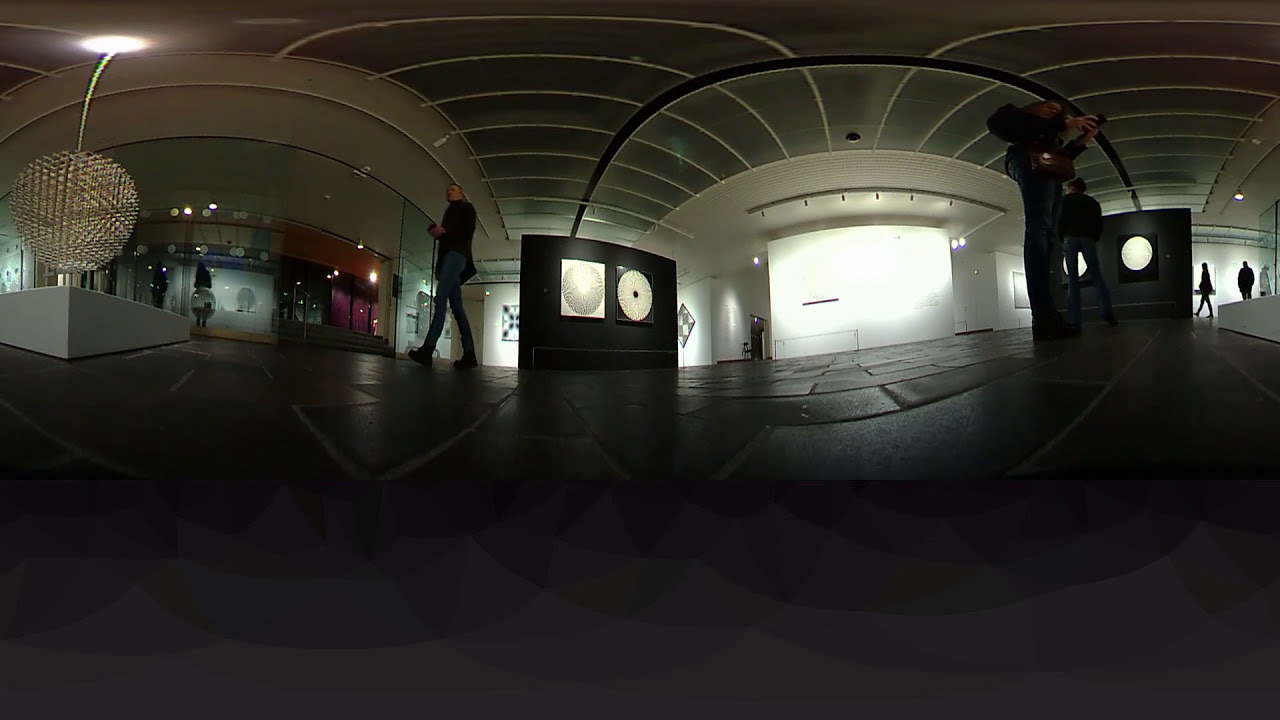This 360-degree panoramic image, likely taken in an art gallery or museum, showcases a dimly lit space where the walls and various pieces of art are the primary illuminated elements. The image suffers from some heavy distortion, making it challenging to discern fine details. In the foreground, a black area suggests a roadway, while further along, a sidewalk is visible with at least three pedestrians.

The gallery features well-dressed visitors, some sporting designer jeans and holding cameras, as they examine the exhibits. Several of the art pieces appear circular in shape, although distortion makes it difficult to be certain. A man in a suit is prominently displayed towards the left, and other figures are seen milling about, including a woman apparently taking a photo and another man gazing intently at a white wall, washed out from strong illumination, giving the impression that he is viewing art, although no specific pieces are discernible there.

One notable sculpture, likely fashioned from a white grid with a green stem, resembles an apple or a cherry and adds to the artistic ambiance of the setting. Additionally, there is a structure resembling a disco ball suspended from the ceiling. Various other installations and pieces of art are scattered throughout the room, contributing to the overall gallery experience. The ceiling, like much of the room, remains in shadow, enhancing the dim and subdued atmosphere.